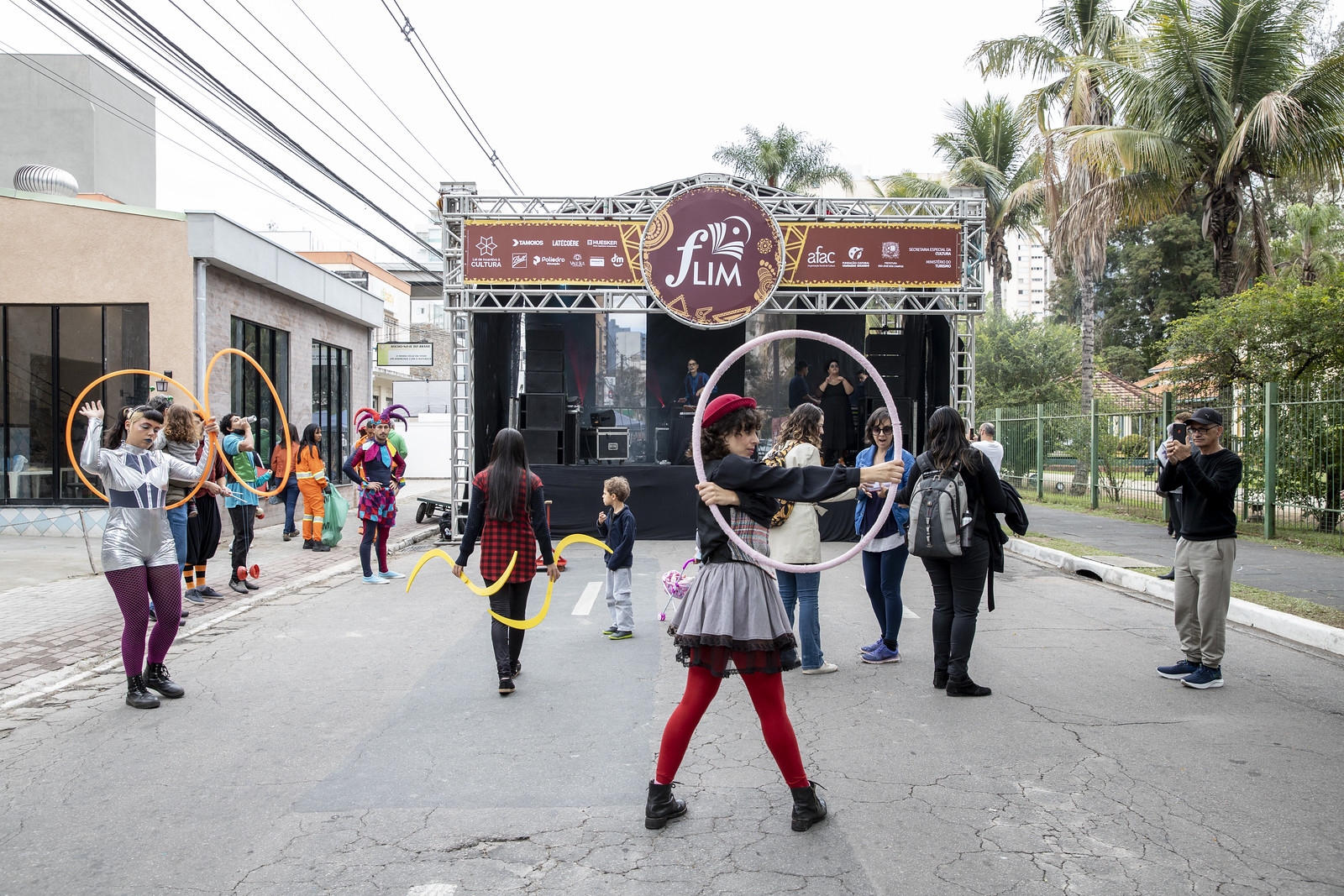In this vibrant outdoor image taken during the daytime, we see a lively street performance featuring several costumed entertainers. The scene is set on a paved street, noticeably cracked, and closed off to traffic for the event. Central in the foreground, a young Caucasian girl, dressed in a black shirt, white skirt over red leggings, and a red hat, holds a hula hoop with her right arm crossed in front of her chest and her left arm extended. Her torso twists to reveal the right side of her partially turned face. Flanking her, several other performers also hold brightly colored hula hoops, including one woman to the left in a silver jumpsuit with purple tights and black shoes. Another woman in a red plaid long-sleeve shirt on the left side holds yellow S-shaped objects. 

In the background, a group of people stands around, including a young child and a man dressed in a black shirt and gray pants capturing the activity with his cell phone. Behind them, a small stage is set up on the street, adorned with amplifiers and a banner displaying the word "FLIM." Buildings line the left side, and on the right, a fence with trees, possibly palm trees, suggests a nearby park. Overhead, the sky is gray, intersected by power lines in the upper left corner. The mood is festive, captured in the colorful attire and dynamic poses of the performers, providing a snapshot of a lively street parade or performance.